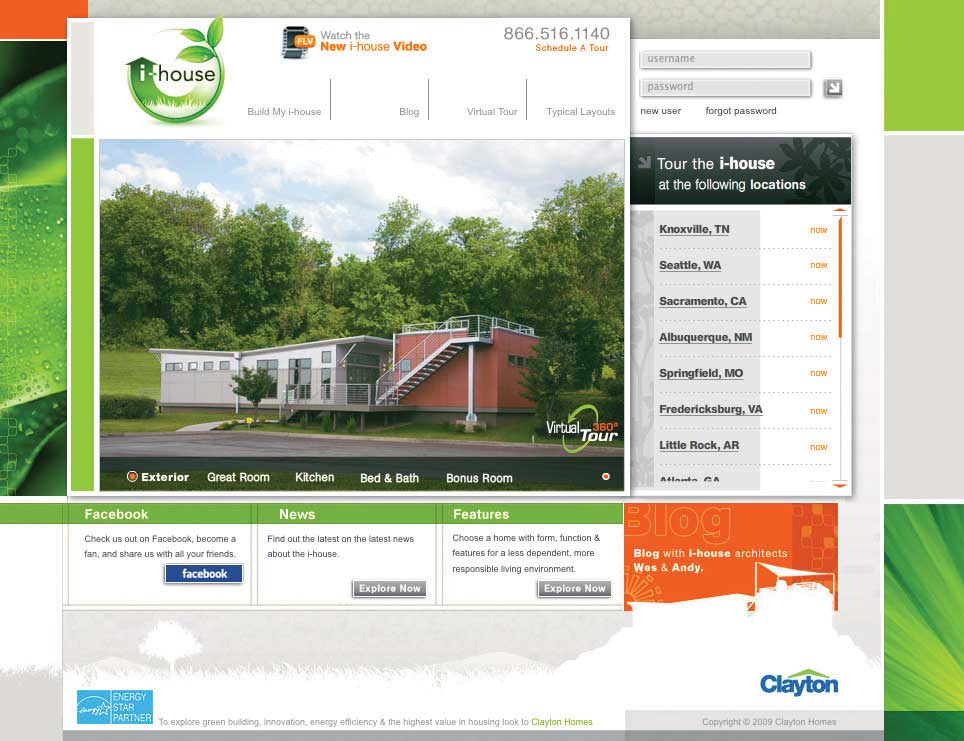Screen capture of the iHouse website. The main focus of the page is an illustration of a stylized house where the roof forms an arrow and branches wrap around it. Prominently displayed are the words "Watch New iHouse Video" next to a contact phone number. Below that, the text invites users to "Tour the iHouse at the following locations" and offers a virtual tour. This tour includes 360-degree views of various parts of the iHouse: the exterior, a living room, kitchen, bedroom, bathroom, and a bonus room. Additionally, the website features links to Facebook, news, features, and a blog, providing multiple ways for users to explore and engage with the iHouse concept. The iHouse itself is depicted as a small, square, manufactured home that can be constructed in a factory and delivered to a customer's yard by truck.